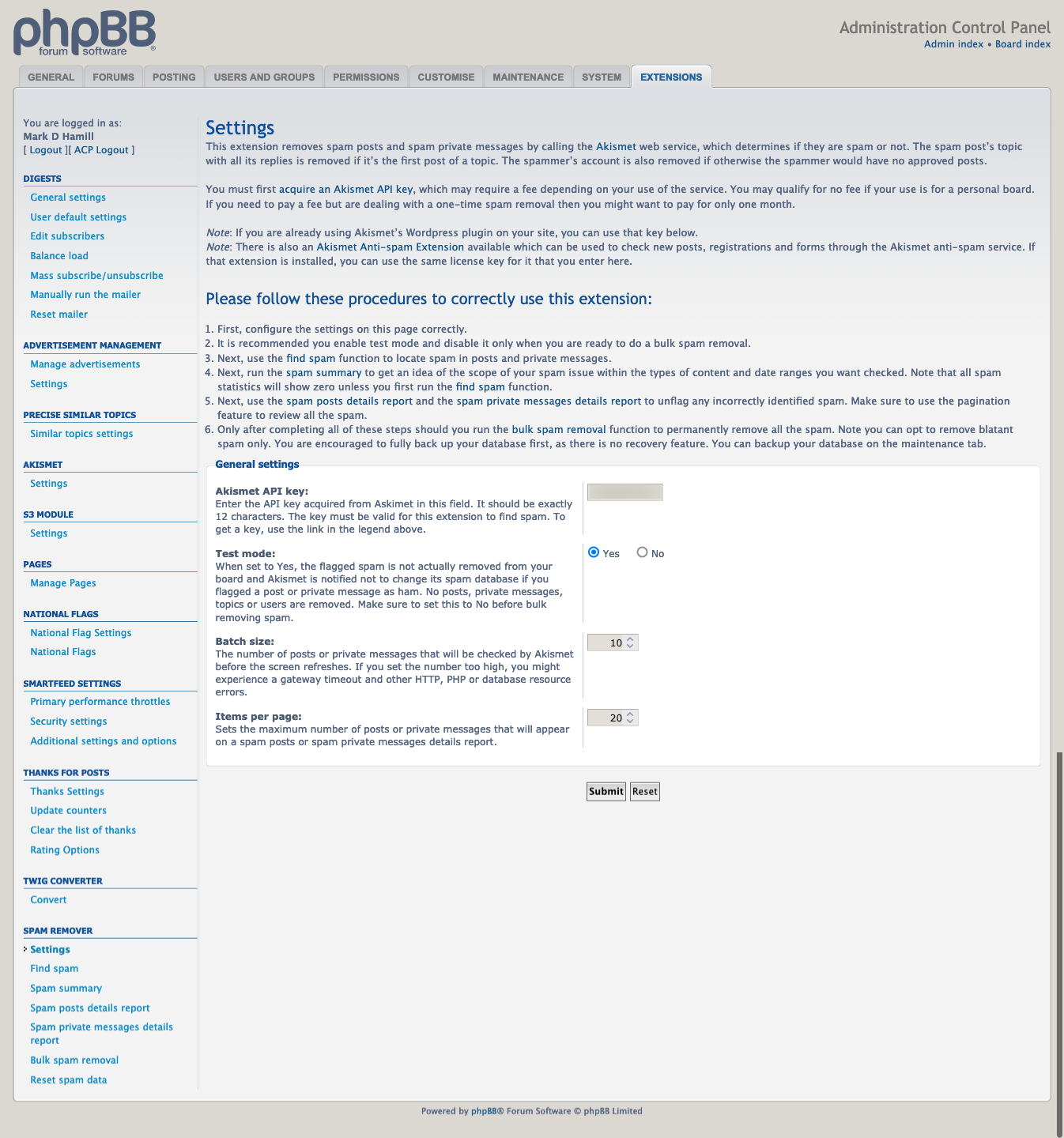The image displays an administration control panel user interface with a tan background. At the top of the panel, in lowercase letters, it says "phpBB," followed by some text too small to discern. On the right-hand side, it prominently displays "Administration Control Panel" with additional, illegible text in blue. 

Below the header, a series of tabs are shown. Most tabs have a grey background, except for the last one, which has a white background. 

Running down the left-hand side, there are numerous words in blue. Some of these words are dark blue and underlined, while others are light blue and not underlined. 

To the right section of the interface, a heading in blue reads "Settings," with several options listed below it. A directive follows: "Please follow these procedures to correctly use this extension," accompanied by a numbered list of instructions. 

Further down, under "General Settings," there is a white rectangular area with several paragraphs on the left and a grey rectangle to the right. Below this grey rectangle, two radio buttons are visible: one outlined in blue with a blue dot inside, labeled "Yes," and another outlined in grey labeled "No." 

Two grey rectangles beneath these buttons contain the numbers "14" and "20" respectively, each accompanied by up and down arrows. Finally, at the bottom of the panel, there are "Submit" and "Reset" buttons.